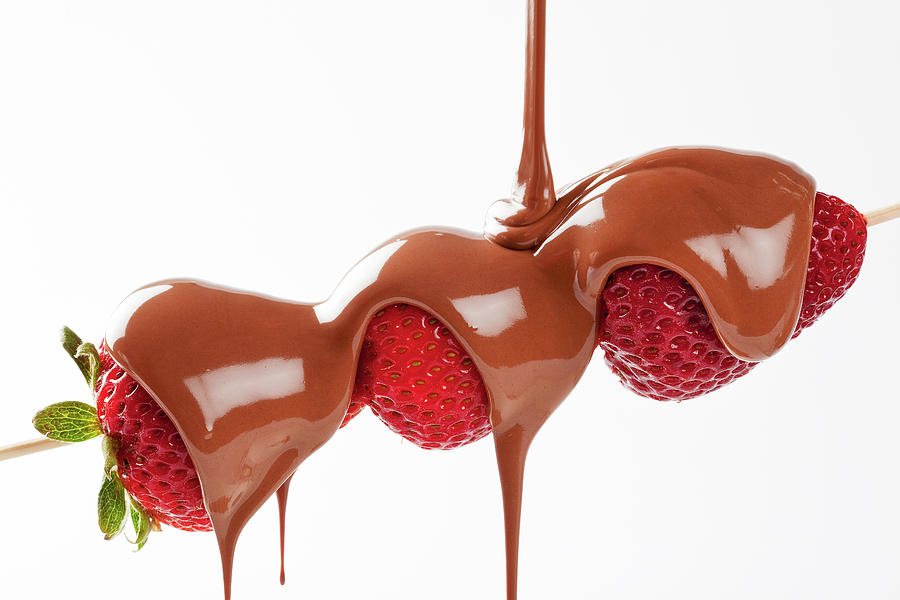A detailed photograph showcases three bright red, ripe strawberries skewered on a stick, against a stark white background. The strawberries are being generously drizzled with a glossy, light brown milk chocolate, streaming from an out-of-frame source at the top of the image. The chocolate gleams under bright lighting, reflecting spots of light as it cascades over the fruit, particularly thick on the topmost strawberry, which uniquely retains its green leaves. The leaves create a vibrant contrast against the rich chocolate, which drips tantalizingly towards an unseen destination beyond the frame. The skewer is visible, poking out from both sides of the strawberries, anchoring the vivid and mouth-watering composition in the center of the picture.